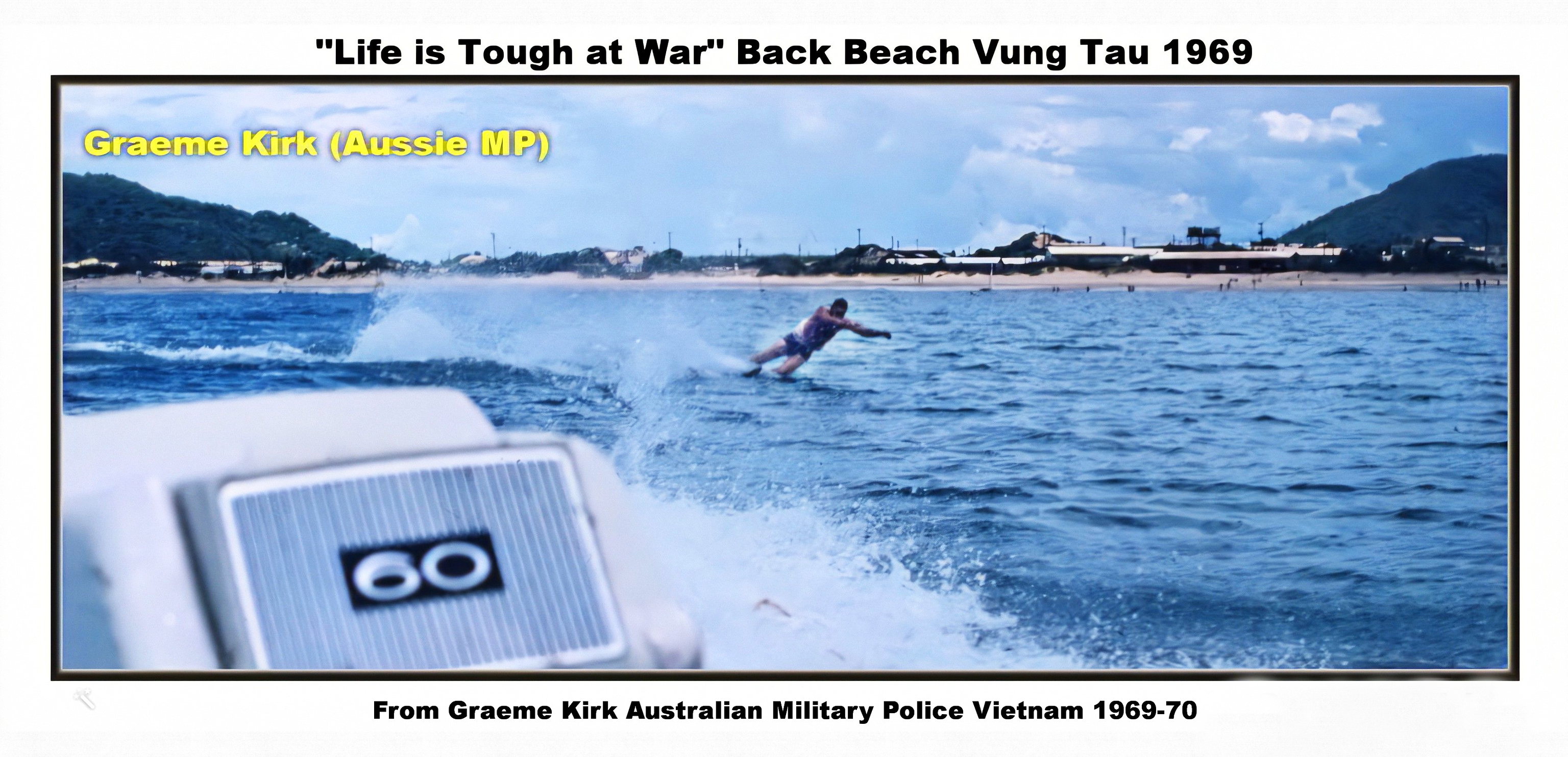This landscape photograph taken in 1969 captures a vibrant scene from the back of a sea vehicle in Vung Tau, Vietnam. The image, bordered in gray with a thin black pinstripe, features the text "Life is tough at war. Back Beach, Vung Tau, 1969" at the top, and "From Graham Kirk, Australian Military Police, Vietnam, 1969-70" at the bottom, in black print.

In the foreground, the bottom left corner of the photograph shows part of the water vehicle, identifiable by the number 60 on its equipment. Central to the scene is a man jumping into the strikingly blue sea, surrounded by an expansive body of water. The scene is set under a broad, partially clouded blue sky, indicating it is likely taken during midday.

In the distance, the shoreline meets gentle hills dotted with some buildings, framing the serene yet dynamic moment captured on film. Written in yellow in the upper left corner is "Graham Kirk" with "Aussie MP" in parentheses, marking the photograph's historical and personal context. The clear, vivid colors of white, gray, black, yellow, blue, and green enhance the detailed richness of this snapshot from the past.